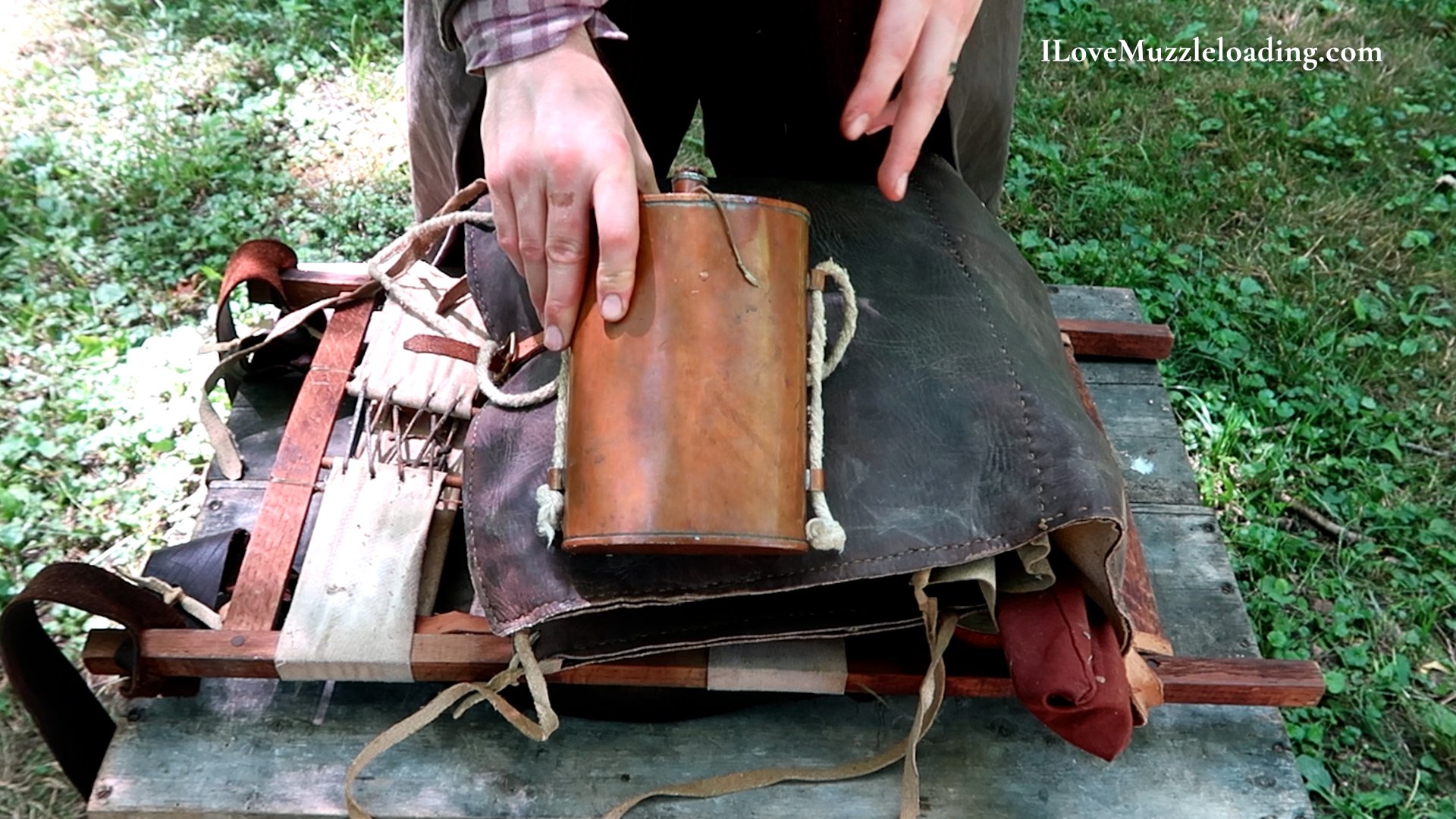In the landscape-oriented color photograph, we see a vivid, detailed scene outdoors. Two white-skinned hands are centrally positioned, each hand appearing twice if not thrice smaller than the massive object they are holding. This large, canteen-like object appears to be a flask made from brown leather, accentuated with white threads on its sides. The flask is so sizable that it dominates the hands' scale, underscoring its humongous nature.

The flask is resting on a dark brown leather tote bag, which in turn is seated atop a wooden frame reminiscent of a washboard. This wooden support features a white fabric band laced at the center, adding intricate detail to the overall composition. Beneath the wooden structure, there appears to be a cement slab.

In the top left corner of the photograph, the white text "ILOVEMUZZLELOADING.COM" is set against a backdrop of green grass, which is a recurring visual throughout the background, framing the scene with natural greenery. The photo captures the tactile variety of leather, wood, cloth, and metal, lending it a richly textured quality that aligns with the style of photographic representationalism realism.